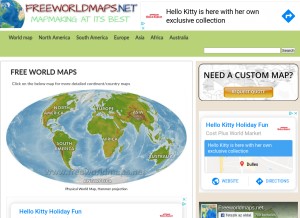The image depicts a small website layout centered around map resources, specifically showcasing an image of a globe. At the top of the page, there is a white banner featuring a partial image of a globe. Prominently displayed in the banner is the website name, "FREEWORLDMAPS.NET," with "FREEWORLDMAPS" in bold, red, uppercase letters and the ".NET" in blue.

Beneath the banner, a tagline reads, "Map making at its best," in a light green font, although the choice of color makes it less legible. At the very center of the page, there is some text in red, but it's too small to make out clearly. The text appears to announce, "Hello Kitty is here with her own exclusive collection," implying that Hello Kitty-themed maps are available.

To the right of this central text, there's a blue diamond symbol with an indiscernible emblem inside. Below these elements, a green navigation bar provides various options for users, including a search bar. The main choices seem to be geographic regions like World Map, North America, South America, Europe, Asia, Africa, and Australia, allowing users to dive into more detailed map selections.

Further down, an image displays the entire world set against a white background, shown in an oval form. To the right of this image, there's a prompt reading, "Need a custom map?" indicating personalized map services are offered. Additionally, there is a clickable option to view the specific collection of Hello Kitty maps.